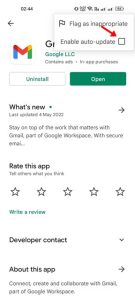A blurry screenshot from a mobile-optimized website prominently features a Gmail installation page. The page displays black text on a white background with various elements slightly obscured due to the blurriness. At the top left, the number "0044" is visible next to some mobile icons, while on the right, a small box with a flag icon is labeled "Flag as inappropriate." An option labeled "Enable auto-updates" is accompanied by a square box with a red diagonal arrow pointing down towards it. Below this, the Gmail logo is partly covered by the elements above.

Two buttons are positioned under the logo: an "Open" button in green on the right and an "Uninstall" button in white on the left, indicating that Gmail is already installed. The section below explains the new features: "Stay on top of work that matters with Gmail, part of Google Workspace with secure email." Additional options include "Rate this app," "Write a review," "Developer contact," and "About the app." Near the bottom, though blurry, there appear to be the words "Connect or convert" and a message encouraging users to "Create and collaborate with Gmail, part of Google Workspace."